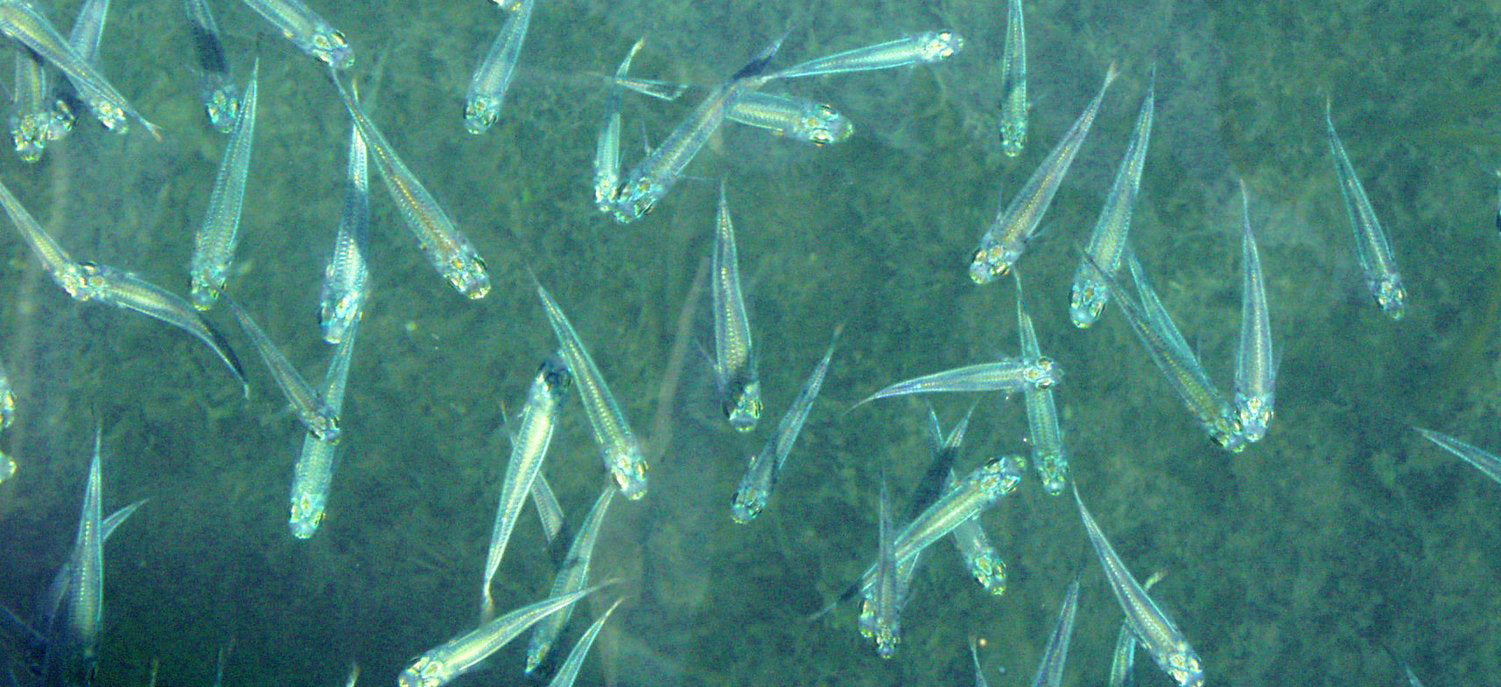The image features a captivating underwater scene teeming with small, translucent fish, resembling minnows, swimming in various directions. The fish, numbering around twenty, exhibit subtle yellow features near their middle, with their outer parts and tails almost clear. They appear to have round faces and elongated bodies, contributing to their delicate, almost ethereal appearance. The background is a mesmerizing bluish-green gradient, with shades of teal, green, and even hints of yellow blending together, evoking the sense of being deep underwater. The setting, likely an ocean or a lake, is devoid of text, allowing the viewer's focus to remain on the multitude of fish and their fluid, chaotic movement. The scene is further enriched by faint, hazy green seaweed, adding to the overall depth and allure of the underwater environment.